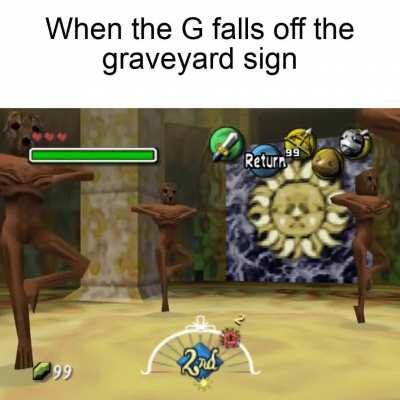This image is a somewhat blurry screenshot from the video game "The Legend of Zelda: Majora's Mask," featuring a humorous meme. The scene appears to take place in an ancient, brownish-gray setting with large square pillars and a cement-colored floor. Central to the joke, the text at the top says, "When the G falls off the graveyard sign," implying a comedic scenario where zombies, resembling dancing creatures, are part of the setting. These zombies have non-human faces and are posed standing on one leg with their arms up and elbows pointed outwards. 

There are three of these creatures: the largest is on the left, a smaller one in the middle background, and another one on the right. To emphasize the video game elements, there is typical Nintendo 64 HUD display. On the upper left-hand side, a green horizontal bar likely represents a power or energy meter, flanked by heart icons. Below this, in the bottom left corner, are white numbers "99" accompanied by a green icon, presumably indicating currency (rupees) or item quantity. The top right corner contains familiar N64 icons, including the return arrows and a sword.

In the center bottom of the image, the word "seconds" is displayed over a blue diamond background, enclosed by a decorative white, flower-like arch. Additionally, there are three red circles on the green bar indicating status information. The background features a sun design surrounded by a gray swirly pattern, completing the ancient, mystical ambiance.